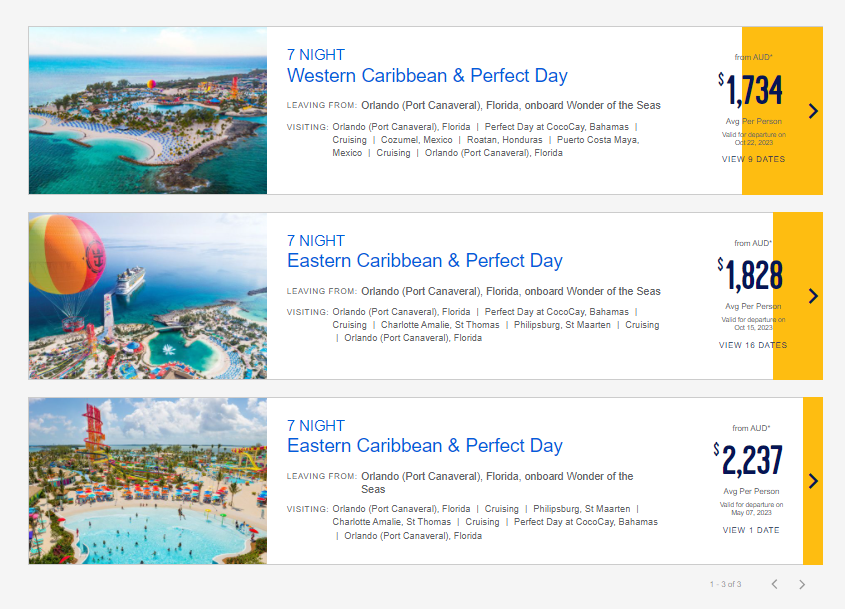This image features a promotional flyer for a Caribbean cruise, segmented into three distinct rows, each illustrating a different cruise package.

In the top section, artistic illustrations depict an idyllic island resort surrounded by pristine waters and sandy beaches. A colorful hot air balloon drifts above this tropical paradise. The caption reads, "7 Night Western Caribbean and Perfect Day," and provides details about the departure point: Orlando, Florida (Port Canaveral), aboard the luxurious ship, Wonder of the Seas. The itinerary includes multiple destinations, and the package is priced at $1,734.

The middle section zooms in closer to the ocean scene, enhancing the visibility of the cruise ship and making the hot air balloon more prominent. This section is labeled, "7 Night Eastern Caribbean and Perfect Day," and is priced at $1,828.

The bottom section offers an even closer view, focusing on a vibrant wave-action pool area, capturing the excitement and activity of the cruise experience. This package is also titled, "7 Night Eastern Caribbean and Perfect Day," but with a higher price tag of $2,237. 

Overall, the flyer effectively conveys a picturesque and luxurious Caribbean vacation, accentuated by the allure of adventure and relaxation.